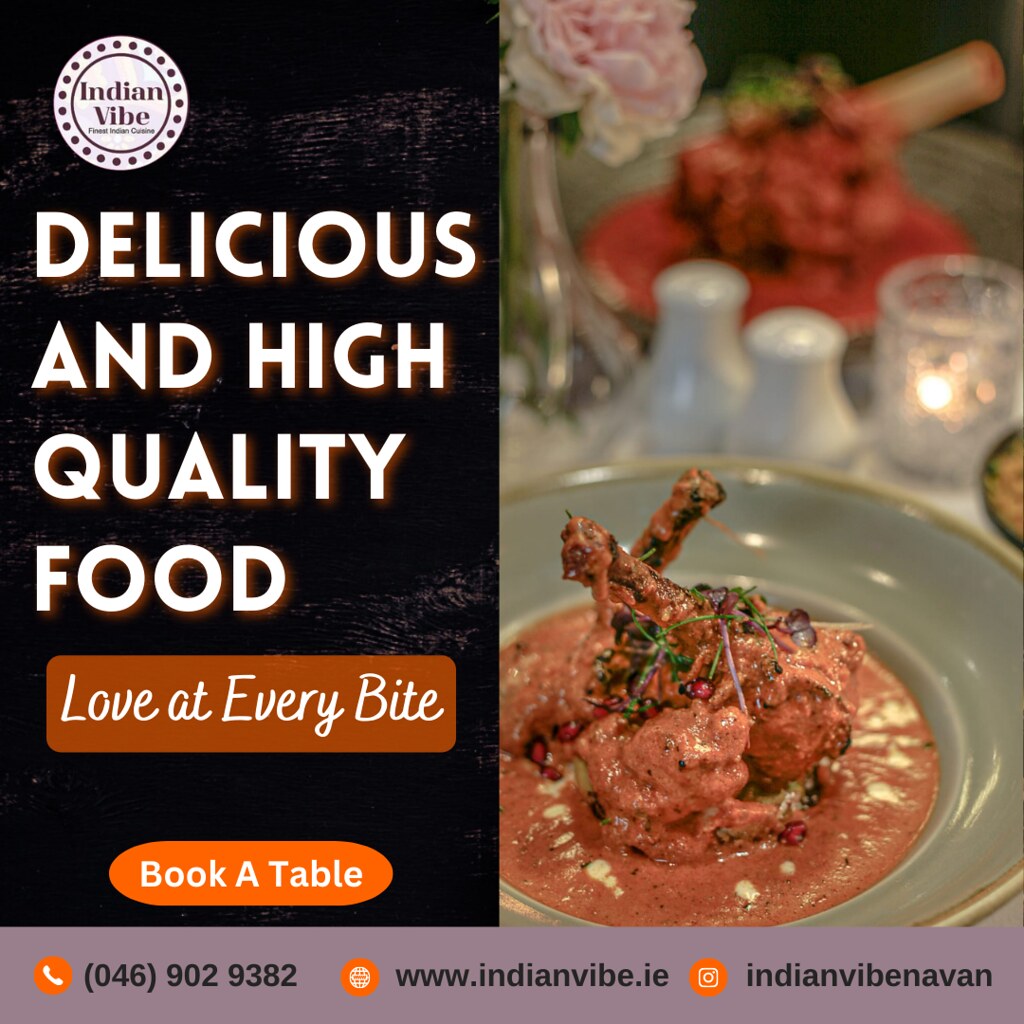The advertisement for the Indian Vibe restaurant features a central, enticing image of a gourmet dish. The dish, displayed on a sophisticated gray plate, appears to consist of tender, pink-hued chicken nestled in a pink yogurt-based sauce, garnished with delicate green and purple strands. Surrounding this centerpiece are out-of-focus elements suggesting a warm and inviting ambiance: salt and pepper shakers, a candle in a glass holder, and vibrant pink flowers. 

On the left side of the image, against a black backdrop, the restaurant's branding is prominently displayed. A circular emblem reads "Indian Vibe," encircled by tiny dots, followed by the tagline "Delicious and High Quality Food" in white text. Below this, a brown box with cursive lettering invites patrons to "Love at Every Bite," and an orange oval button encourages them to "Book a Table." 

At the very bottom, a purple banner provides essential contact details: a phone number (046-902-9382), a website (www.indianvibe.ie), and a likely social media link indicated by a camera lens icon. These elements together convey a sophisticated and appetizing snapshot of the Indian Vibe dining experience, emphasizing both quality and accessibility.